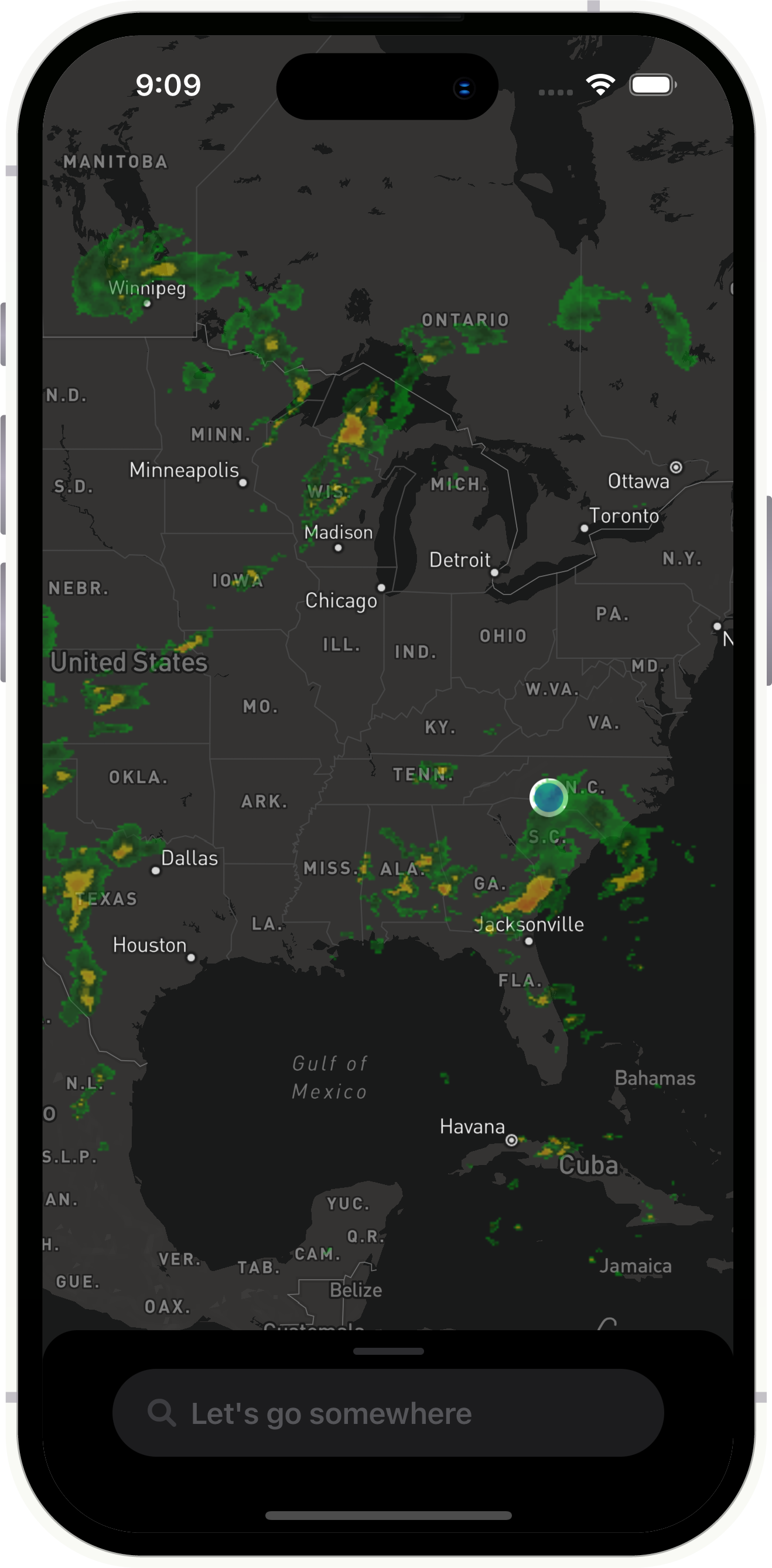The image displayed on the screen captures a weather app showcasing an extensive radar view covering the central United States extending eastward, encompassing parts of Canada including Ontario, Manitoba, and Winnipeg, as well as reaching south into the Gulf of Mexico and Cuba. The backdrop of the map is black, with land areas represented in a dark gray hue. Water bodies are shown in black. A teal dot is prominently positioned between North Carolina and South Carolina, which might indicate the current location of the user. The radar reveals various weather systems, predominantly in green, signifying areas of rain. Lesser but noticeable patches of yellow, orange, and red indicate more intense weather activity, potentially signifying heavier rainfall or storm development.